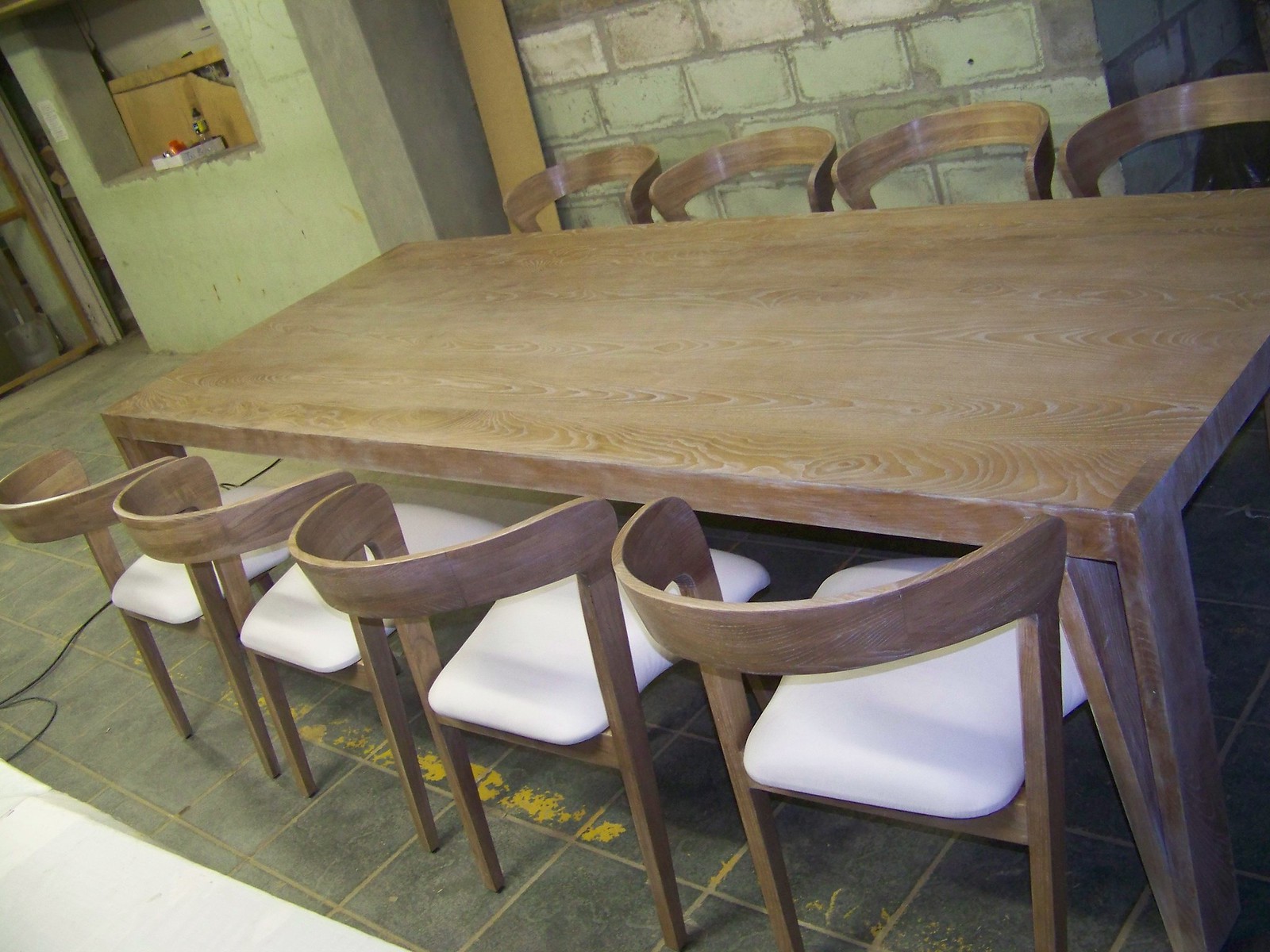This color photograph presents a rustic yet modern indoor setting, featuring a large rectangular wooden dining table with eight matching wooden chairs, organized in a landscape orientation. The table is aligned lengthwise towards the camera, flanked by four chairs on each side. Each chair has an arched back designed to fit the contour of a seated person's back, with noticeable white cushions on the seats, providing contrast and comfort.

The floor beneath the table is covered in dark gray tiles with interspersed black accents, and the grout lines appear to be dirty brown or yellow, hinting at age or wear. Notably, some patches of yellow, either from wear or paint splatters, are visible under the table. A prominent black cable runs from left to right across the floor, adding to the room's unfinished aesthetic.

Behind the dining arrangement is a brick wall with large, lime-green breezeblock-style bricks and beige areas that fade into the background. Signs of weathering and repairs are visible, with grey mortar touch-ups adding to the distressed charm. On the right-hand side, the brick wall stretches into the background at a 90-degree angle.

To the left of the table, part of another wall can be seen with a square opening containing a white box topped with something red. An additional entrance way and green-tinted wall sections are also partially visible, enhancing the room's eclectic and unfinished vibe.